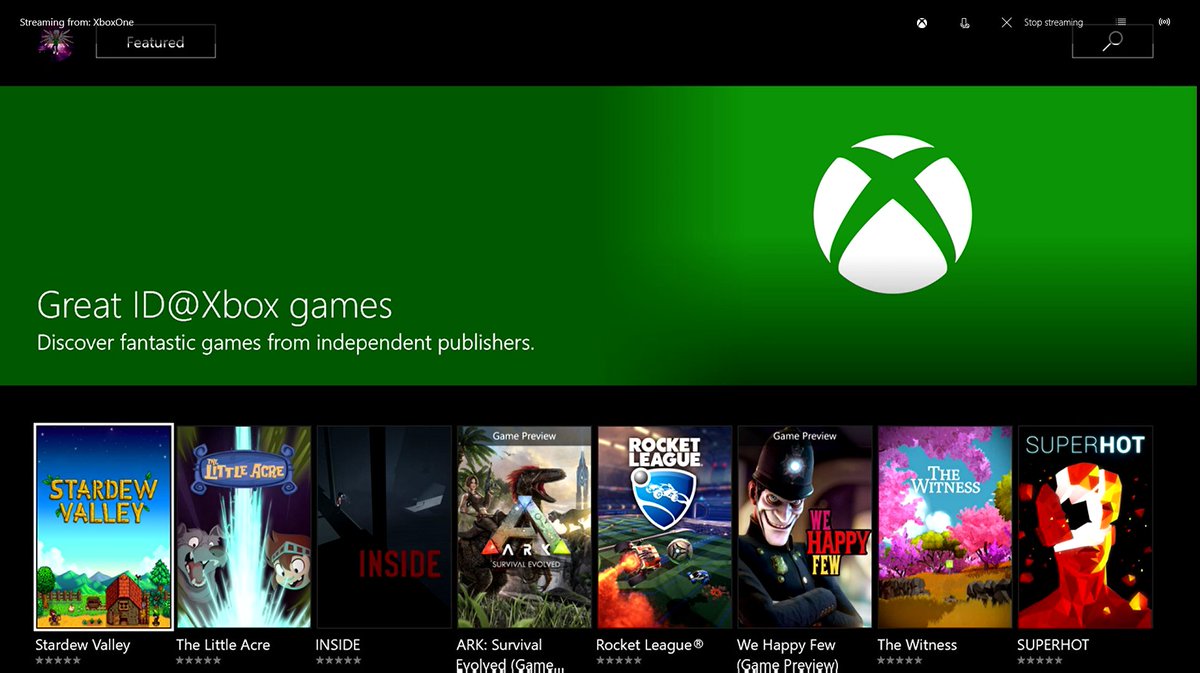The image is an advertisement for Xbox. At the top left corner, it features a black header with an Xbox logo, accented by a hint of purple, alongside various icons. Below the header, there's a search bar for users to explore content. Centrally, a vivid green section displays the headline: "Great ID@Xbox Games," followed by the tagline, "Discover fantastic games from independent publishers." 

Beneath this text, a collection of eight Xbox game covers is lined up, each bursting with vibrant colors and unique visuals:

1. **Stardew Valley** - The cover is adorned with a starry sky, emphasizing its serene, countryside setting.
2. **The Little Acre** - This cover is animated, showcasing its charming and whimsical art style.
3. **Inside** - A dark and eerie cover, shrouded in heavy shadows, hinting at its suspenseful and atmospheric nature.
4. **Ark** - Features an animated depiction of a dinosaur, highlighting its adventurous gameplay and prehistoric themes.
5. **Rocket League** - Sports-themed cover showcasing high-octane cars, indicating competitive and fast-paced gameplay.
6. **We Happy Few** - Displays an animated police officer looking down with a smile, suggesting an unsettling, dystopian narrative.
7. **The Witness** - Showcases a tranquil, outdoor scene with trees adorned with pink flowers, lush grass, and rolling landscapes, reflecting its puzzle-solving elements.
8. **Super Hot** - Highlighted by a starkly contrasting red figure set against a minimalist black and white backdrop, signaling its intense and distinctive gameplay style.